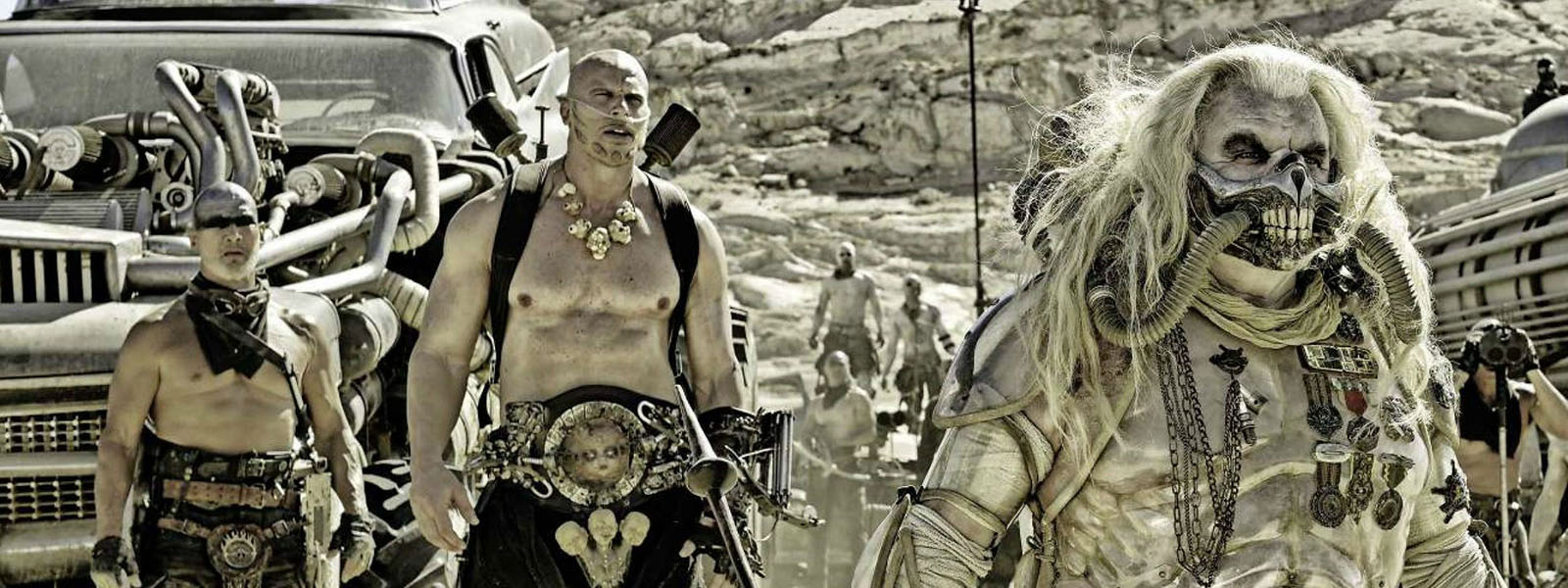In this striking and detailed still from the movie "Mad Max: Fury Road," the scene is set in a sun-drenched, post-apocalyptic desert landscape that evokes the iconic, washed-out aesthetic of the film. Dominating the foreground on the right side is a menacing figure, the warlord who presides over the bandits hoarding precious water. He is distinguishable by his skull-like mask with painted teeth and a complex breathing apparatus, juxtaposed against his long, flowing white hair and a silver, armored bodysuit adorned with metals. Flanking him over his right shoulder are two muscular, shirtless men, embodying the brutality of the warrior tribe, who stand vigilant and poised. The background reveals a chaotic tableau of more bandits, bare-chested with grotesque and monstrous features, brandishing weapons. They are surrounded by large, imposing vehicles with exposed engines, adding to the scene's intense and raw energy. The backdrop is completed by rocky hills, bathed in the blazing sunlight, enhancing the harsh and unforgiving nature of their world.